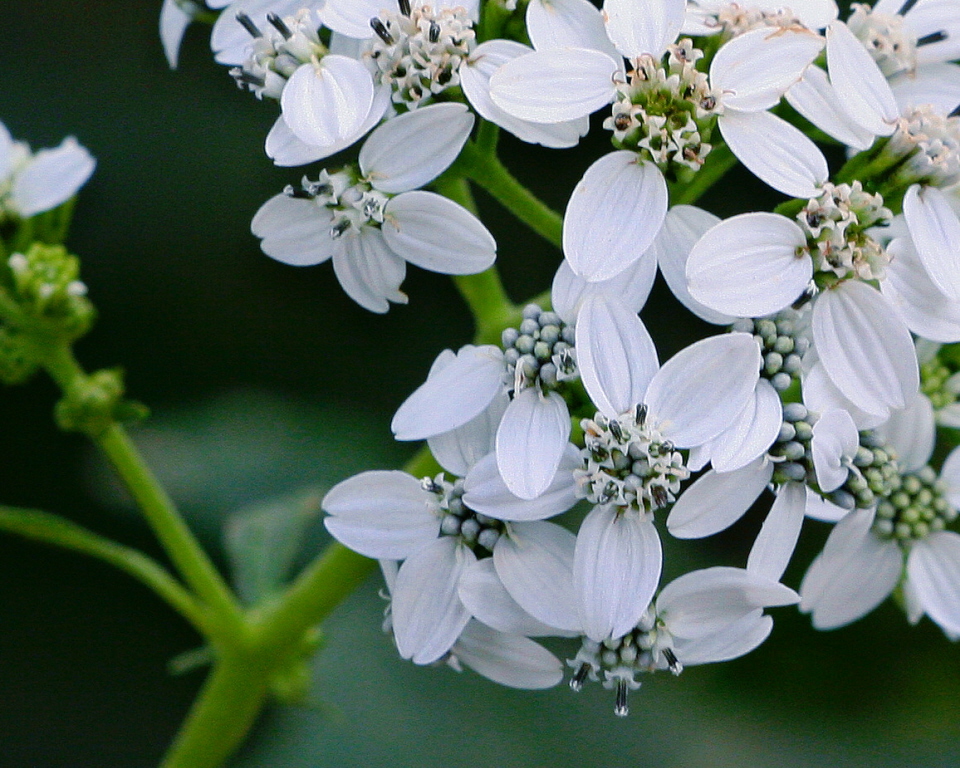This close-up image captures a cluster of blooming dogwood flowers (or a similar species), characterized by their distinctive white petals, typically numbering four to six per flower. Each bloom features a central collection of small, round, green buds that resemble berries, which are also flowering. The bright green stem, appearing slightly out of focus, runs diagonally across the image from the lower left corner towards the upper right corner, with additional sprigs extending upward. The composition prominently displays the flowers from the center to the top right, with some stems visible through the petals. The background is dark and blurred, enhancing the sharpness and brightness of the floral cluster, while a subtle patch of green is noticeable at the bottom of the frame.